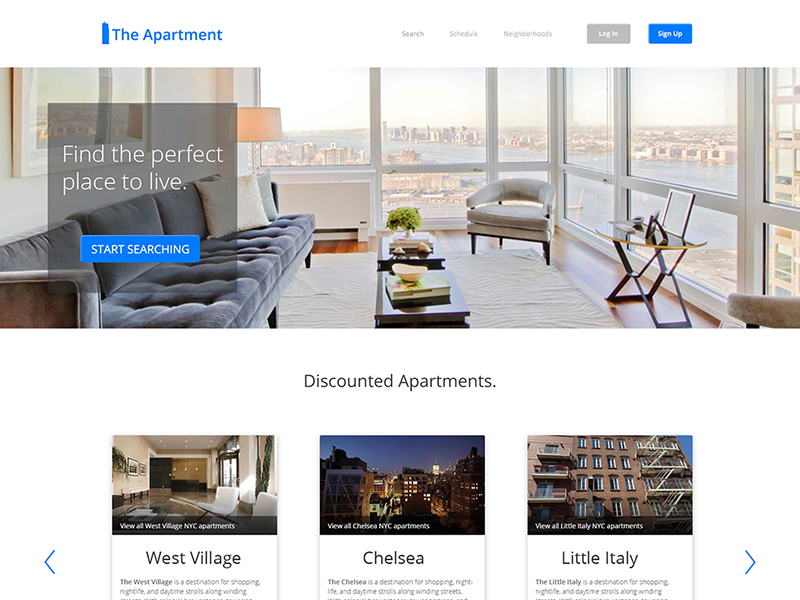The screenshot captures a webpage for an apartment search service called "The Apartment." The page features a clean, white background with various sections for navigation and information.

- **Top Section**:
  - The title "The Apartment" is displayed in blue text.
  - Below, in gray text, options like "Search," "Schedule," and "Neighborhoods" are listed.
  - To the right, there is a light blue button with white text that says "Login," and a dark blue button with white text that says "Sign Up."

- **Main Image**:
  - The central image is a modern apartment with large windows on all sides, separated by white framing. The view from the apartment showcases a serene river and a cityscape in the background.
  
- **Left Sidebar**:
  - A gray box contains the text "Find the perfect place to live" in white and blue. Below, there is a blue button with white text that reads "Start Searching."
  - Additional gray text beneath the button mentions "Discounted apartments."

- **Featured Neighborhoods**:
  - The names "West Village," "Chelsea," and "Little Italy" are listed, suggesting a focus on New York City neighborhoods.
  
- **Navigation Arrows**:
  - Gray arrows are present on both the left and right sides for further browsing.
  - There is small, unreadable text beneath some images, likely describing the city or specific listings.

Overall, the page provides a user-friendly interface to explore apartment options in notable neighborhoods, especially within New York City.